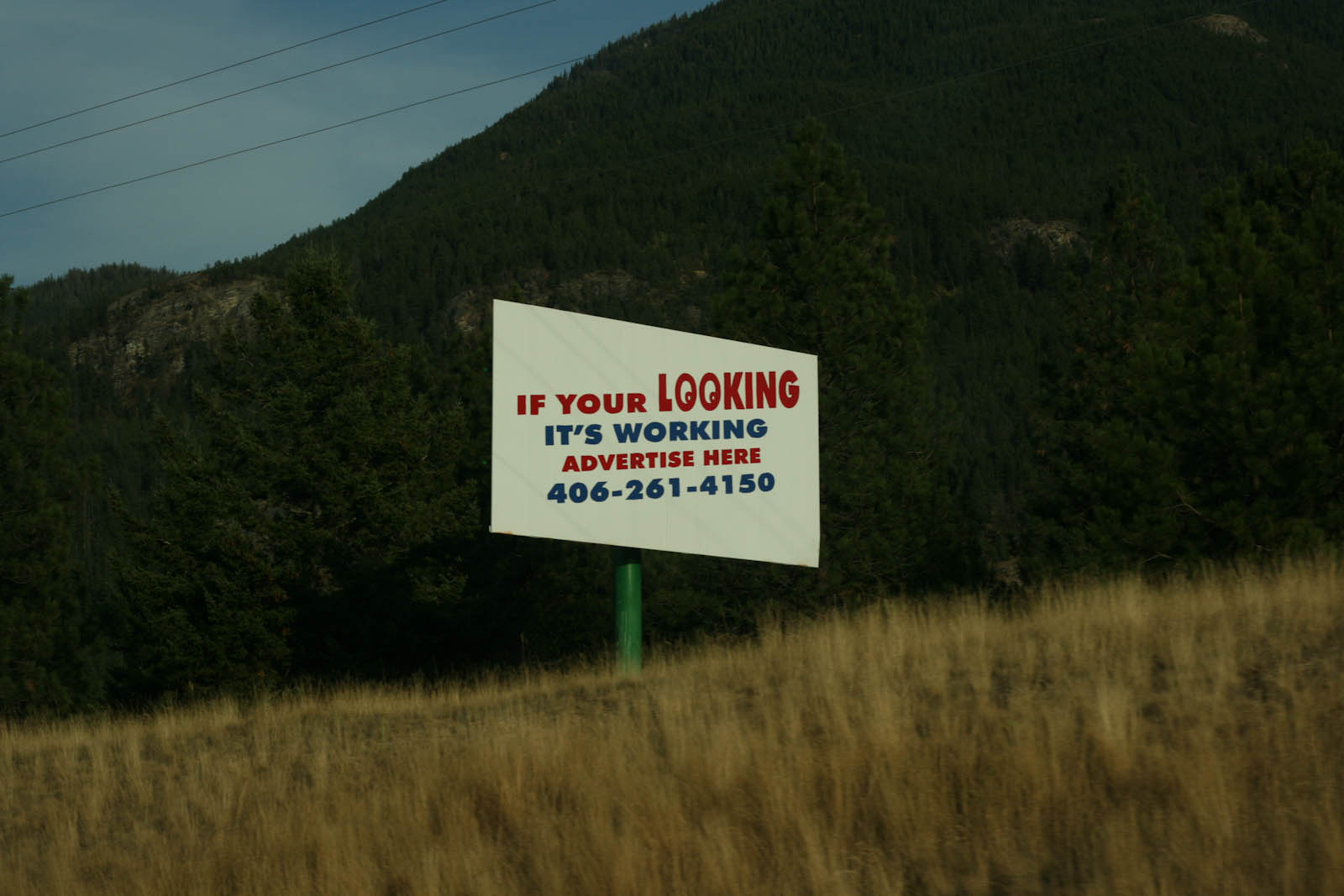In this photograph, a billboard stands prominently in an open field. The foreground is covered with dried, brown grass, adding a rustic touch to the scene. The background is lush with dense tree cover in various shades of dark green, interspersed with noticeable rock outcroppings. Overhead, the blue sky peeks through, contrasting against a few stark, black power lines that traverse the top of the image.

The billboard itself is mounted on a sturdy green post and features a white background. The text on the billboard is eye-catching, with a playful, marketing twist. In bold red font, it reads "If you're looking," where the two 'O's are designed as googly eyes, drawing immediate attention. Below, in a contrasting blue font, it states, "It's working." Further down, the red-font text encourages, "Advertise here," followed by a contact number in blue font: 406-261-4150. The billboard's design skillfully uses color and playful typography to convey its message effectively.